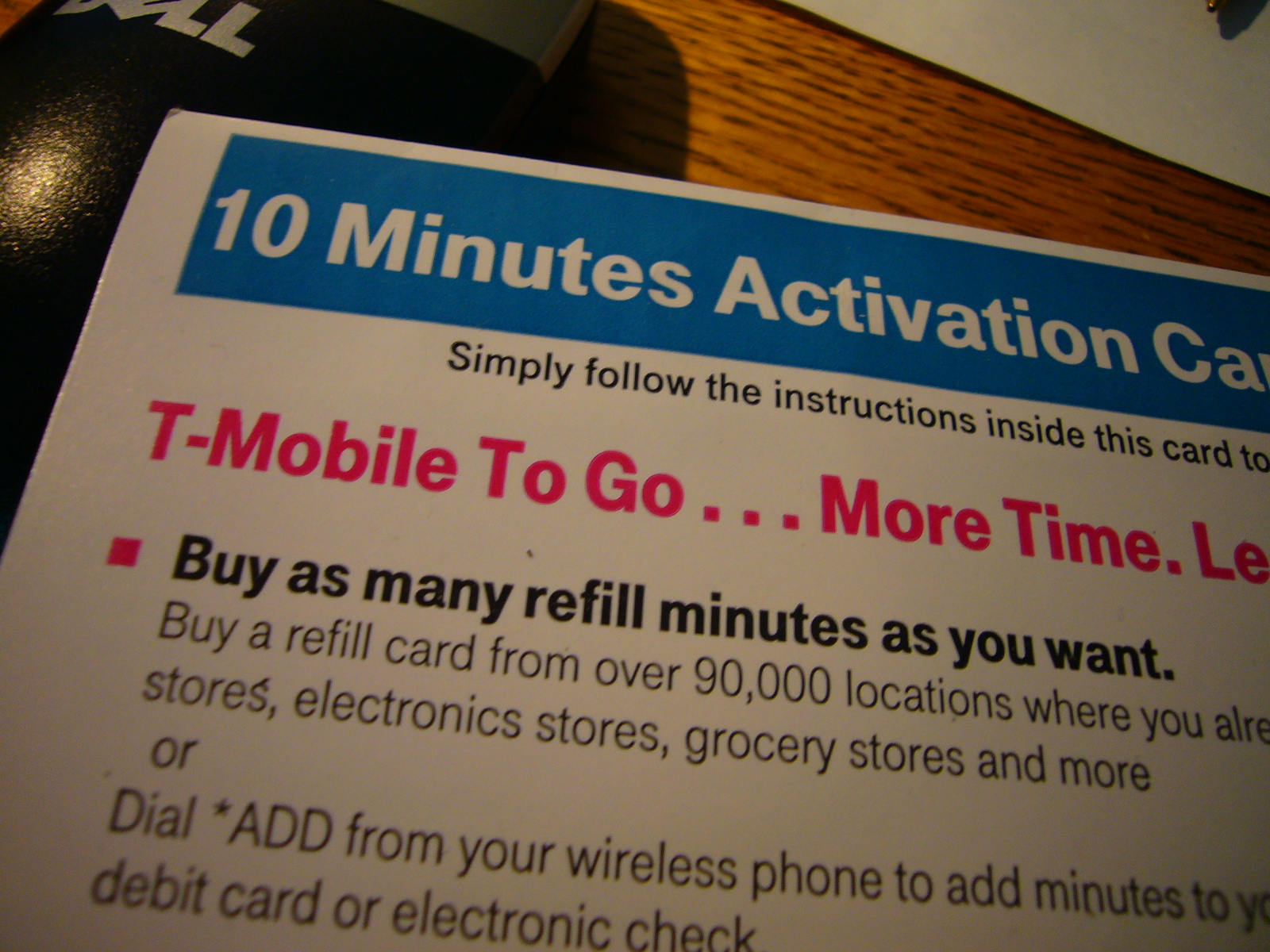The close-up image features a T-Mobile activation card, prominently displaying a blue horizontal border at the top with white text that reads "10 minutes activation card." Beneath this, there are instructions in black text advising to "simply follow the instructions inside this card." The pink text below states "T-Mobile to go more time," although some of the wording is cut off. The black bullet point below that specifies, "buy as many refill minutes as you want," followed by directions to purchase a refill card available at over 90,000 locations such as electronic and grocery stores, or to dial ADD from your wireless phone to add minutes using a debit card or electronic check. The card is slightly tilted clockwise, with its upper left corner resting on a Dell-branded computer mouse, all placed on a wooden table. The visible sections of the wooden table surround the card and mouse, and there’s a blue section with white letters at the top indicating "ten minutes activation card," but some parts are obscured due to the cropping of the image.